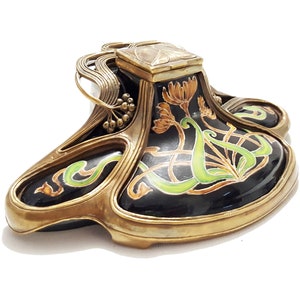The image depicts a highly ornate, irregularly round-shaped Japanese figurine that combines elements of both furniture and decorative art. The figurine features a rounded bottom with three rounded edges that taper into the center, ascending into a distinct square top. The entire piece is outlined in lavish gold detailing. The flat top of the figurine acts as a lid, adorned with a small gold tree-like structure that extends outwards, with small balls attached at its ends.

The main body of the figurine is decorated with a black background, against which vibrant orange flowers with green stems are painted. These stems extend across different sections of the figurine, connecting various black areas. The black regions are accentuated with floral designs in multiple colors, including green, gold, orange, and brown, lending a richly detailed and intricate appearance to the piece. The design is further elaborated with gold, string-like objects that curve and wind around the floral motifs, creating a melting, flowing effect.

Overall, the intricate and vibrant detailing, along with the combination of rounded and square shapes, make this figure a striking example of ornamental craftsmanship.